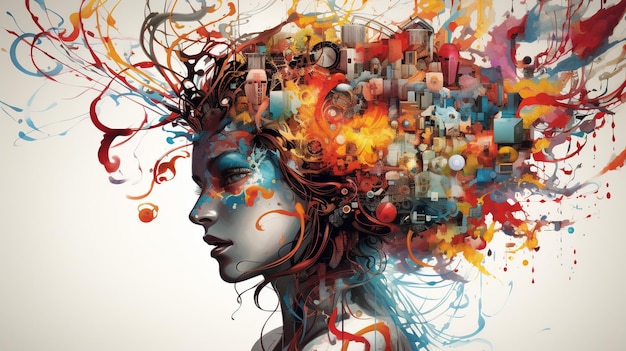The hyper-realistic landscape artwork portrays a young woman with ashen, whitish-grey skin. Her face is black and white, with dark red lipstick adorning her slightly open lips. She gazes intently into the distance, her expression serene yet contemplative. The background features a similar whitish-grey tinge, blending seamlessly with her complexion.

Remarkably, instead of hair, vibrant, multi-colored paint splatters emanate from where the back of her head would be. These splashes of color cascade in all directions—predominantly backwards to the right, but also downwards across her shoulders and upwards to the left. The vivid swirls of red, blue, grey, orange, pink, and turquoise create an explosive crown, symbolizing a creative outpouring. Within this kaleidoscope, discernible shapes suggest buildings and other abstract forms, representing the intricate workings of her mind and imagination. This bohemian and artistic depiction captures the essence of unleashed creativity, vividly illustrating the abstract thoughts and ideas swirling within her consciousness.